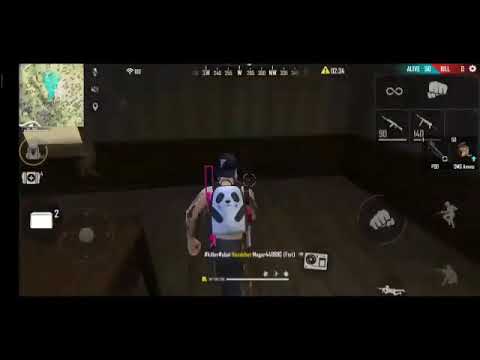The image is a highly detailed screenshot of a third-person video game, possibly Fortnite, capturing a scene within a room that features wooden floors, walls, and a table. The central character, seemingly controlled by the player, appears to be a Caucasian male adorned in a sleeveless shirt and dark pants. He is equipped with a distinct panda-themed backpack displaying a panda face and arms, alongside two rifles strapped on either side, one notably pink. The character wears a backward cap and a motorcycle-style helmet. The comprehensive heads-up display includes a mini-map in the top left, a compass at the top center, and various icons displaying health, weapon selections, and inventory details. On the right-hand side of the screen, there are touch interface buttons indicating actions like punching, crouching, crawling, or jumping, suggesting that this might be a mobile version of the game.